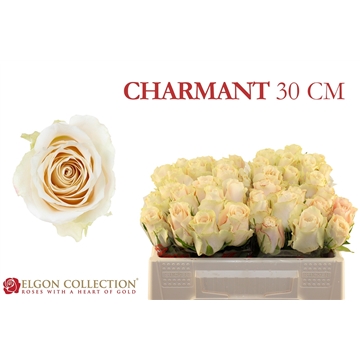The advertisement image features a white background with prominent elements. At the top right-hand corner, in bold red capital letters, it reads "CHARMANT 30 CM." On the left-hand side, there is a single white rose, viewed from above, showcasing a circular pattern of petals. Below this rose, in the bottom left corner, is the distinctive red rose logo paired with the text "ELGIN COLLECTION - Roses with a Heart of Gold," written in a golden-colored font. To the right of the logo, occupying the bottom right section of the image, is a square grayish box containing several roses of a matching yellowish-gold shade, viewed as if looking directly at the box rather than from above. This cohesive presentation suggests an elegant advertisement for the Charmant 30 cm collection under the Elgin brand.